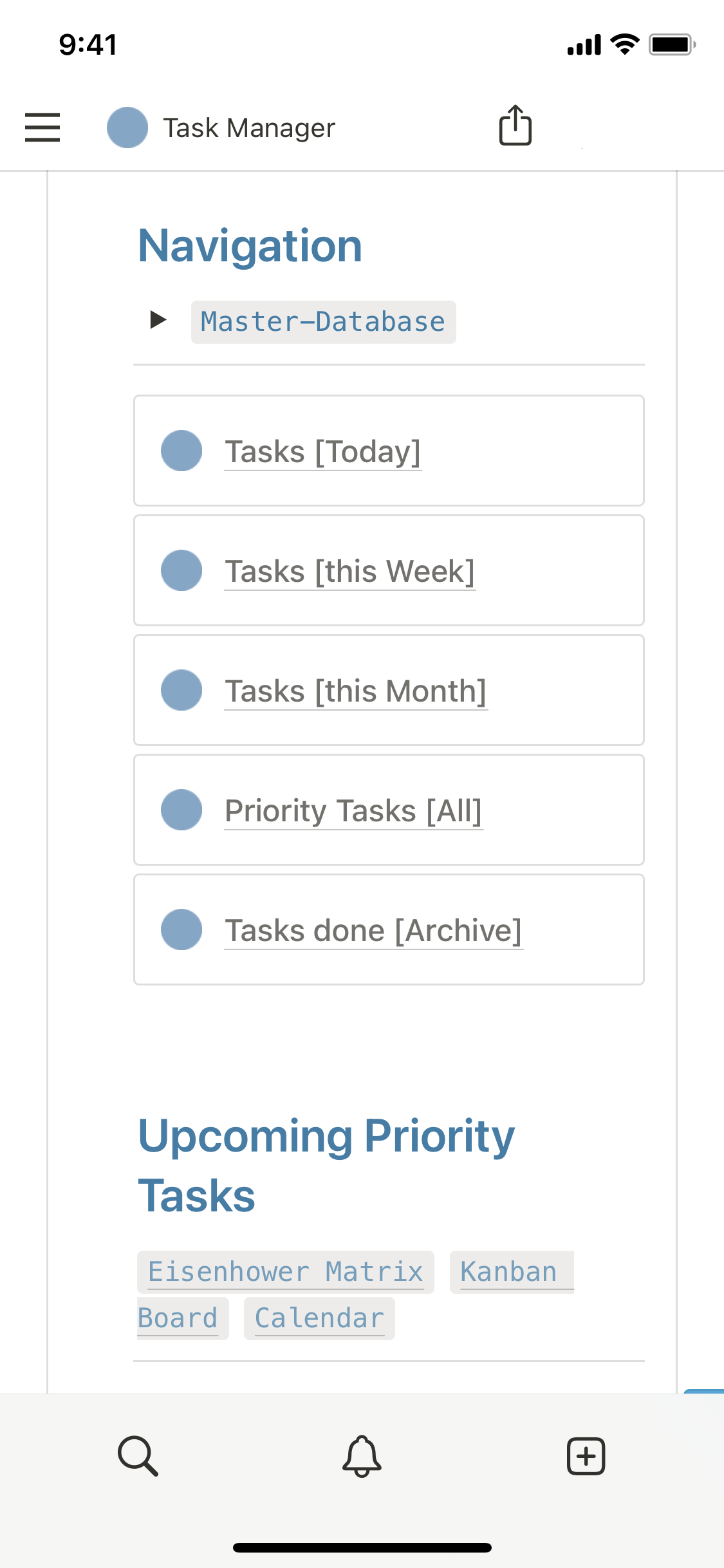The image depicts a smartphone screen displaying the time as 9:41 PM, shown in the top right corner. In the upper left-hand corner, the screen indicates a strong internet connection with four bars and a fully charged battery. Below this, there is a hamburger menu icon alongside a blue button labeled "Task Manager" and an option to download it. 

Further down, the screen features a light blue navigation header with a sizable font. Beneath this, a button labeled "Master Database" is present. Aligned below the header are five interactive options, each accompanied by a blue clickable button. The options listed from top to bottom are:

1. Task (Today)
2. Task (This Week)
3. Task (This Month)
4. Priority Task (All)
5. Task Done (Archive)

After these options, there is a skip, followed by large blue text reading "Upcoming Priority Task." Under this section are four choices, each within a clickable gray rectangle. The options are listed as follows:

- Eisenhower Matrix
- Combine
- Board
- Calendar